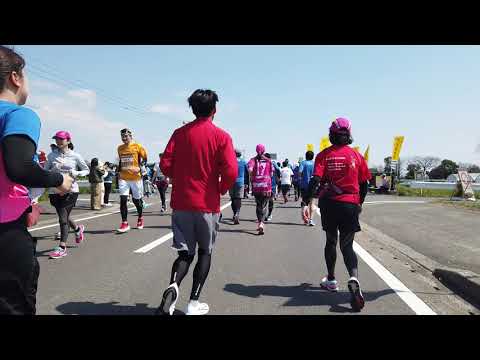This photograph captures a lively scene of an organized foot race on a paved city street, possibly outside of America, given the demographics of the runners. The race course is demarcated by a gray pavement road with white markings on the sides and a dashed white line down the middle, separating the lanes for runners. Competitors on the left side of the road are running towards the viewer, while those on the right side are running away, creating a dynamic and bustling atmosphere. 

In the foreground, the runners' attire is vividly detailed: a young man in a long-sleeve red shirt, gray shorts, black leggings, and white sneakers, and an older Asian woman in a pink baseball cap, red T-shirt, black shorts, black leggings, and white sneakers can be seen. They appear to be running away from the camera. Meanwhile, three or four participants are visible on the left side, running towards the camera.

Spectators line the left side of the road, clapping and cheering the runners. The environment is accented with yellow signage and vertical rectangular yellow flags on the right side. The race unfolds under a mostly clear, light blue sky with a few wispy white clouds. The scene captures the energy and community spirit of a marathon with participants proudly donning various colors such as red, black, yellow, pink, and blue shirts, as well as shorts and high socks. Buildings and trees subtly frame the race, evoking a cityscape on a sunny day. The image also features black horizontal bars at the top and bottom, adding a letterbox effect to the overall composition.